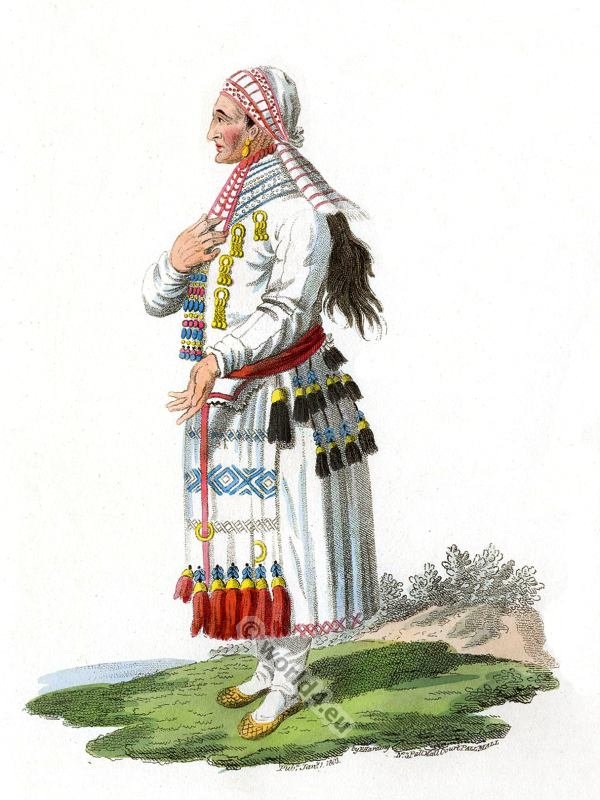This image depicts an older Native American woman standing on a patch of grass, with a simple white background broken by some rocks, greenish plants, and possibly a bush on the right side. The ground below her has a small body of water on the left side. She is dressed in a traditional outfit, comprising a white robe or dress adorned with blue and turquoise, and a red waistband. Her headdress, a thin white and red bandana, ties into a knot and drapes down her neck, complementing her long black hair that appears tied in a ponytail. She wears golden jeweled earrings and red lipstick, enhancing her dignified appearance. Her chest is decorated with various designs, including four pieces of gold jewelry arranged vertically and a scarf featuring a bluish-red circular pattern. At the bottom of her dress, red and black feathers adorn her outfit. Her footwear consists of yellow, scaley-patterned, no-lace shoes. There is a rotated watermark near her heel, indicating the source as "world4.eu," with a copyright icon included.